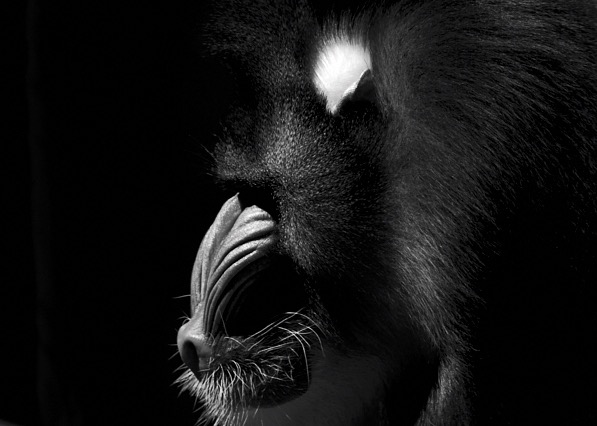In this striking black-and-white photograph, a side profile of a monkey, potentially an orangutan, emerges from total darkness. The background is pitch black, creating a stark contrast with the softly illuminated figure of the monkey. Positioned slightly left of center, the monkey's nose points to the left. The textured nose is long and light gray, with intricate striations and a visible, flared nostril at the tip. Below the nose, a black chin adorned with little white hairs is visible. Just above this, white whiskers sprout from both sides of the mouth and cheeks. Towards the crown of its head is a prominent white spot, while the rest of the monkey's head, back, and arms are covered in straight, bushy black fur. The side of its head reveals a white ear, and although its eyes are obscured by shadows, the fur overhanging its head adds to the creature's mystique. The image is cropped such that the monkey's body extends off the right side of the picture, covering the entire height of the frame. The bottom of the frame cuts off just below its nose, leaving its arm visible only up to just below the shoulder.